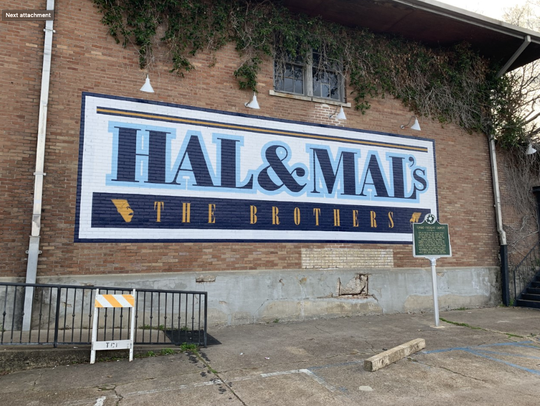The image depicts a detailed mural on the side of a brick wall of a residential-like building. The bricks are visible and unpainted, with windows located above the mural. The mural occupies a significant portion of the wall and features the text "Hal and Mal's" in black writing with a blue highlight around it. Below this, a blue box with yellow writing spells out "The Brothers." A historical marker placard, colored green, stands in front of the building. To the left of this placard, there is a ramp with a black railing, against which a small caution sign leans. The ground in front of the building is a concrete surface with worn-out paint, and there are parking spaces, including a handicapped spot to the far right. The scene suggests it is midday and set in a parking lot, with various colors present, including brown, white, green, light blue, dark blue, tan, orange, and yellow. The center of the image is dominated by the mural, while the top left features text that reads "Next Attachment," and there are plants cascading from the roof, partially covering the upper window.